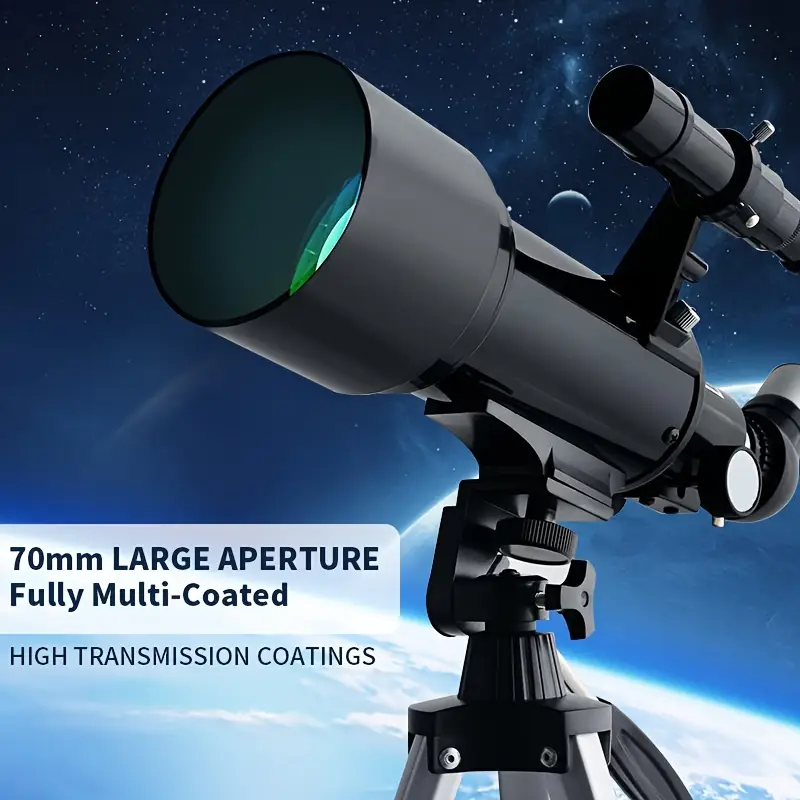Beneath a stunning night sky that transitions from deep black to medium blue with countless stars scattered across the heavens, a crescent moon glows near the top right corner. Dominating the foreground, a sleek black telescope, accented by a hint of blue inside its barrel, rests on a sturdy tripod that gleams in black and silver. The telescope is aimed upward through an eyepiece on its right, guiding the gaze into the celestial expanse. On the left side of the image, a white banner prominently displays the text "70mm LARGE APERTURE" in bold black letters, with additional details below, reading "Fully Multi-Coated" and "High Transmission Coatings," emphasizing its advanced features and the precision it brings to stargazing.